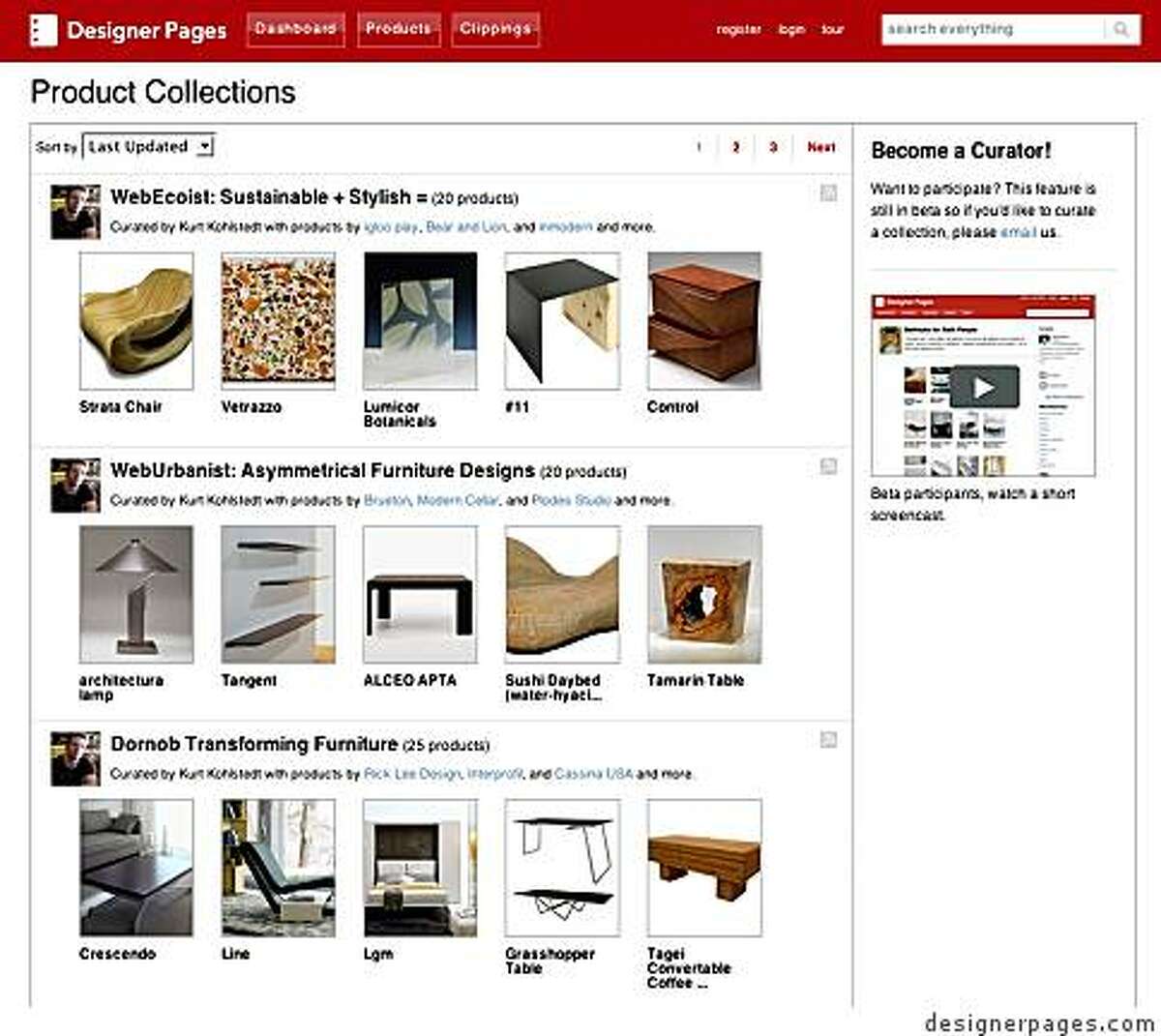The image is a screenshot of a webpage with a predominantly white background. At the top, a brick-red menu header spans the width of the page. On the far left within this header, "Designer Pages" is written in a clean white font. Directly to the right, there is a small white square containing three tiny red rectangles aligned on the left side.

Next to this icon, the menu items are listed in a slightly fainter white font: "Dashboard," "Products," and "Clippings." On the upper right corner of the header, there's a white search box with the placeholder text "Search everything" accompanied by a magnifying glass icon.

Below the header, on the left side of the page, the section "Product Collections" is prominently displayed. This section features a dropdown menu for sorting collections, with "Last Updated" currently selected.

The page showcases various curated furniture collections. The first collection titled "Web Ecoist - Sustainable + Stylish" includes 20 products and is noted to be curated by an unnamed user. Within this collection, there are five thumbnail images: a hardwood dresser, a uniquely designed table, and three other pieces of furniture.

Beneath this, the "Web Urbanist - Asymmetrical Furniture Designs" collection is displayed, also featuring 20 products and similarly curated by an unspecified user. Thumbnails in this collection include a stainless steel lampshade lamp among other modern designs.

Further down, another collection named "Dor Nlb - Transforming Furniture" is mentioned with 25 products. The thumbnails in this collection show versatile furniture pieces, including one that resembles a pool table and another labeled "Grasshopper Table," which appears to feature folding legs.

On the right side of the page is a sidebar starting with an invitation to "Become a Curator!" This section encourages users to participate in curating collections and notes that the feature is still in beta, providing an email address for interested participants. The overall quality of the image is not very good, with some text appearing blurry and hard to read.